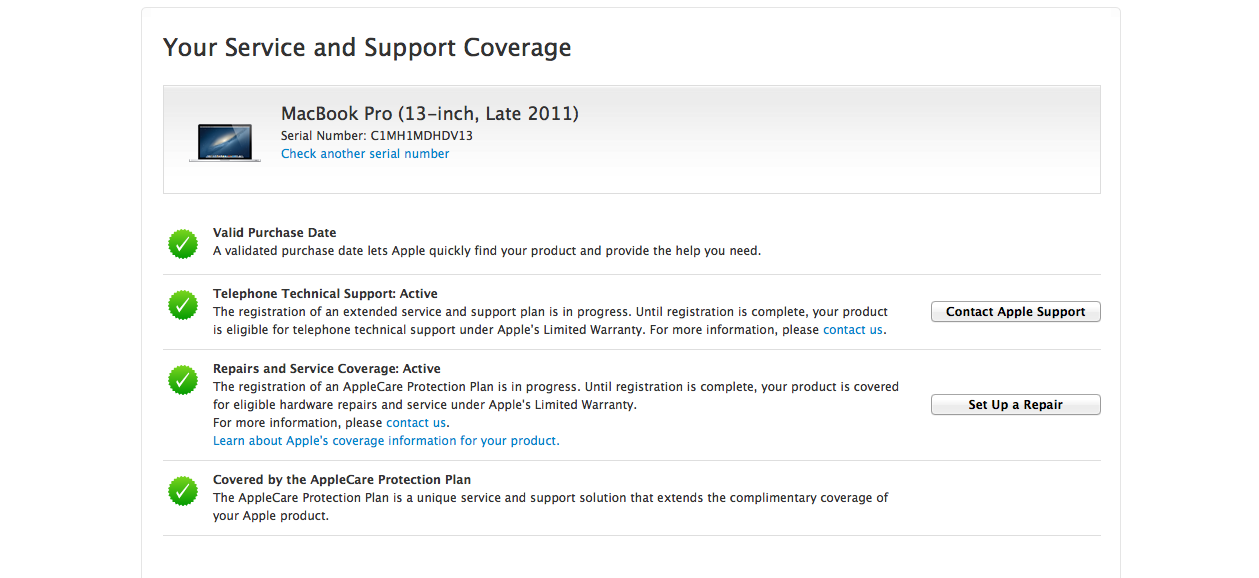This image is a detailed screenshot from a website showcasing the service and coverage plan for a MacBook Pro 13-inch, late 2011 model. At the top, in black text, it says "Your Service and Support Coverage." Directly below, it lists the device model and its serial number (C1MH1MDHVD13), with an option in blue to "Check another serial number." The image has a white background and features four green circles with white check marks, each accompanied by a description in black text:

1. **Valid Purchase Date**: A validated purchase date lets Apple quickly find the product and provide the necessary help.
2. **Telephone Technical Support Active**: Telephone technical support is currently active; the registration of an extended service and support plan is in progress.
3. **Repairs and Service Coverage Active**: Repairs and service coverage are active, and the product is eligible for hardware repairs under Apple's limited warranty.
4. **Covered by the AppleCare Protection Plan**: The device is covered by the AppleCare Protection Plan, which extends the complimentary coverage.

To the right-hand side of these descriptions, there are two buttons labeled "Contact Apple Support" and "Set Up a Repair," both in black font on a white background.